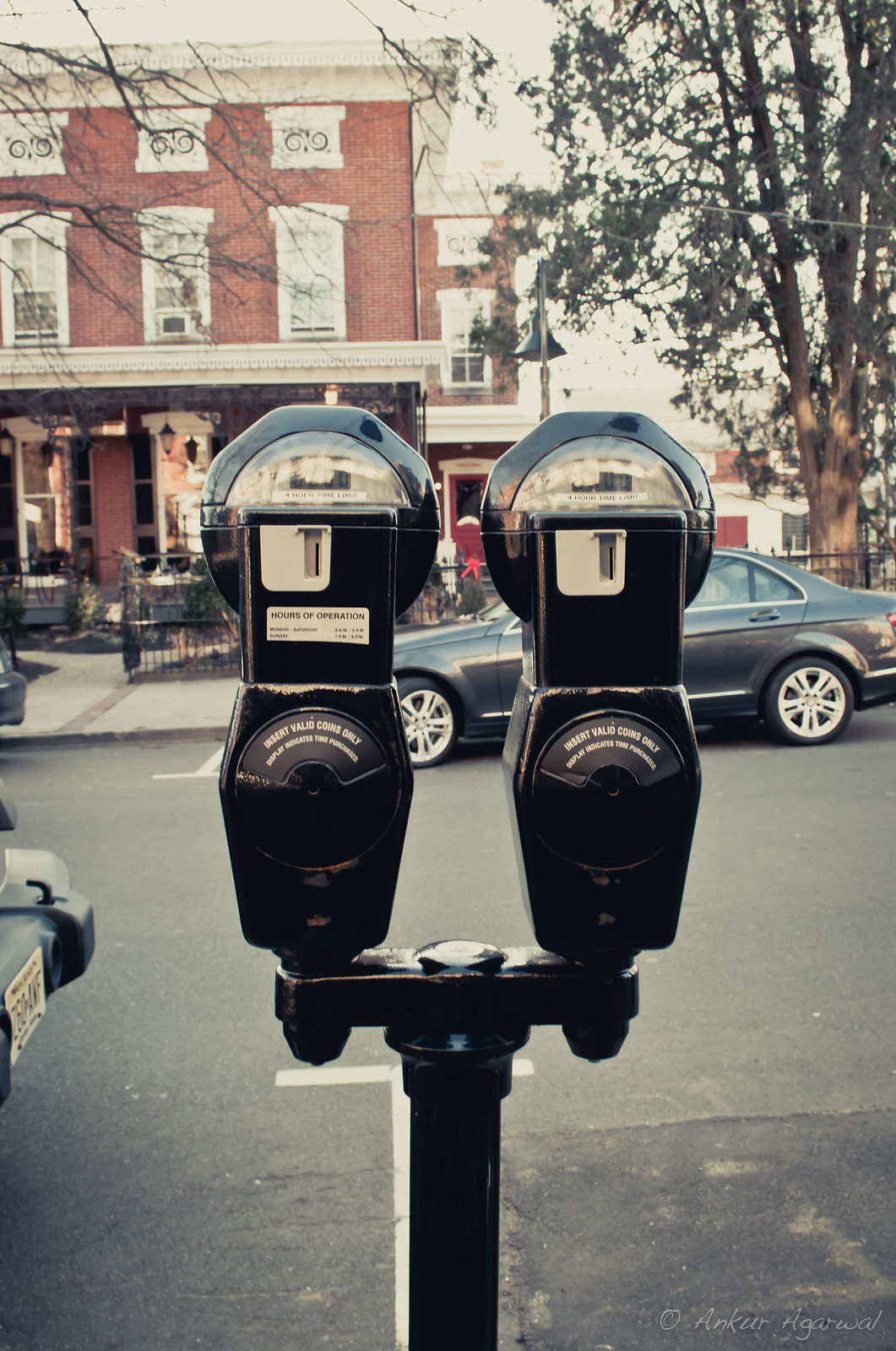This vertically oriented, low-saturation yet sharp and vividly colored artistic photograph captures a close-up of two old-style, black parking meters mounted on a single post, which splits near the top, with each meter featuring a glass semicircular viewing area. The meters, exhibiting distinct metal brushing and wear, stand prominently in the foreground. Open to a four-hour time limit, the meters have inscriptions including "hours of operation" and "insert valid coins only." To the bottom left, a portion of a car bumper with a visible license plate adds contextual depth, while another car, a grey sedan, appears slightly out of focus in the background, parked on the opposite side of the street.

The backdrop reveals a brick brownstone building with windows, a gated area, and a patio, likely part of a city establishment. A tree with leaves partially obscures this building in the upper right corner. The worn texture of the pavement further enriches the scene. The photographer’s signature, bearing a copyright symbol and the name "Ankur Agarwal,” is stamped at the bottom right-hand corner, marking this as a thoughtful piece of urban street photography.